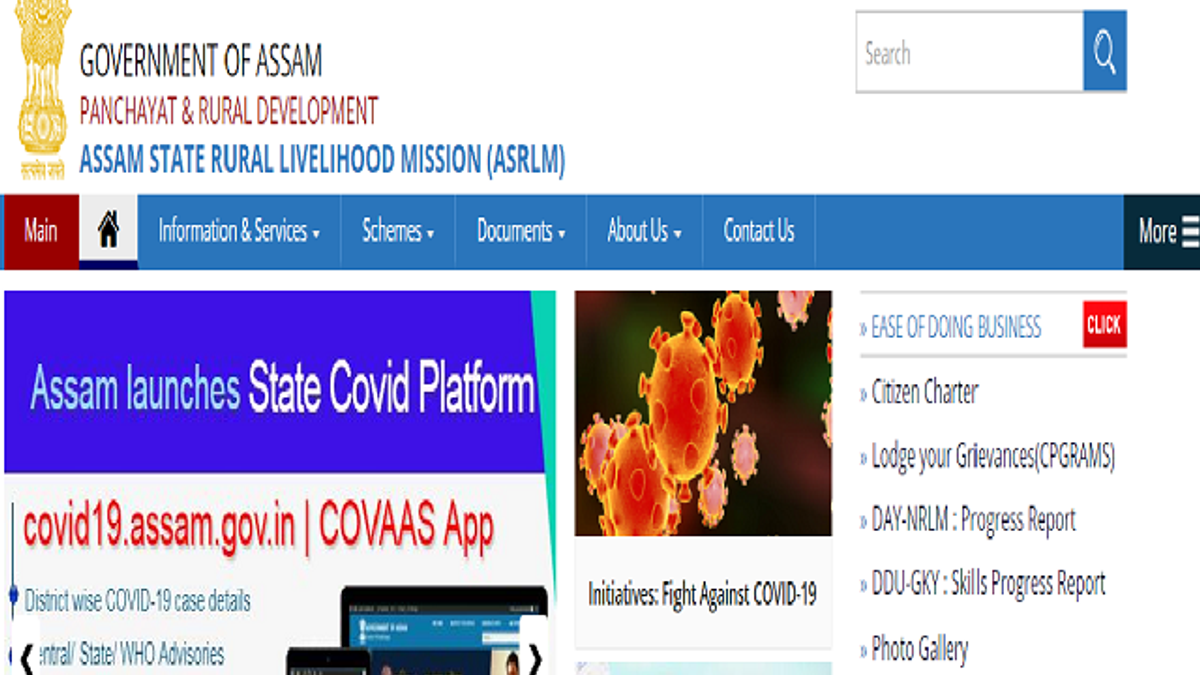The screenshot depicts the homepage of a governmental website with a clean, white background. In the top left corner, the text "Government of Assam" is prominently displayed in a black font. Directly below this, "Panchayat and Rural Development" is written in a red font. Further down, "Assam State Rural Livelihood Mission" is presented in a blue font. Adjacent to this text is an elegant gold emblem resembling a vase.

Below these headers, a blue navigation menu spans across the width of the page, featuring options in white text: "Information and Services," "Schemes," "Documents," "About Us," and "Contact Us." 

On the left-hand side of the page, beneath the header, is a purple rectangular banner announcing "Assam Launches State COVID Platform." Below this announcement, the web address "COVID-19.assam.gov.in" is highlighted in red font, alongside the "COVAS app."

To the right of this banner is a detailed, microscopic image of the COVID-19 virus, depicted as spherical particles with red spike-like nodules on their surfaces.